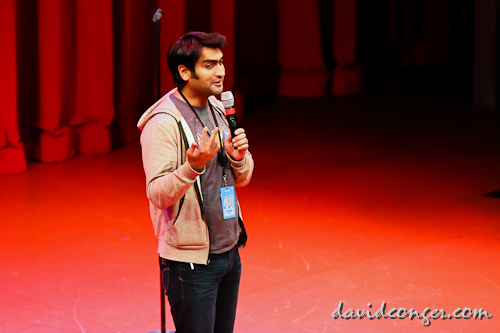In the image, comedian and actor Kumail Nanjiani is standing on a stage with a red-pinkish floor and a backdrop of red curtains. He is dressed in a beige hoodie over a grayish-purple t-shirt, and dark blue jeans. A lanyard with a black rope and a light blue rectangular card, displaying the number 40, hangs around his neck. Kumail holds a black microphone with a red stripe in his left hand while looking off to the side, and his right hand is raised mid-gesture, possibly emphasizing a point. The stage setup includes a podium equipped to hold a microphone. In the bottom corner of the image, there is text reading "davidkansen.com," likely indicating the photograph's source.